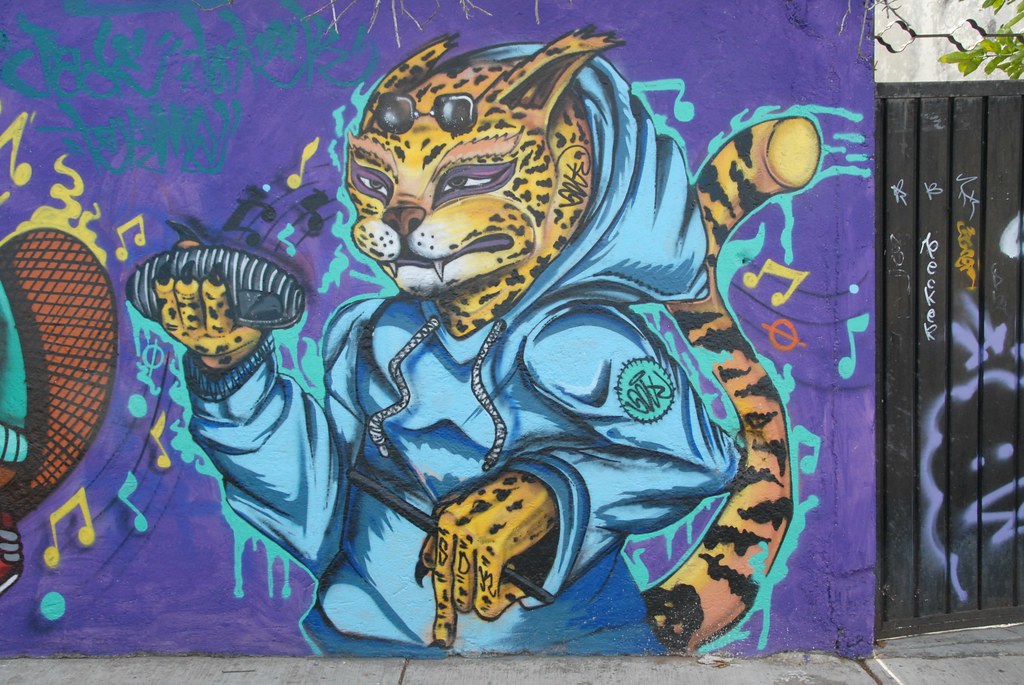In this vibrant photograph, an attention-grabbing piece of street art adorns the side of a purple building. The image captures a small portion of the sidewalk in front of the building, contributing to the urban atmosphere. To the right of the main structure, a black fence or gate, covered with graffiti lines and tags, adds to the city's edgy character.

The centerpiece of the artwork is a striking depiction of a leopard, anthropomorphized and dressed in a light blue hoodie, which is casually pulled up but slightly falling back. The leopard, orange with prominent stripes and a tail, has a cat-like face, complete with sunglasses propped atop its head. Adding another layer of intrigue, the fingers of the leopard feature tattoos that spell out "BDM." In its paw, the leopard is carrying a speaker, emphasizing a musical theme. The background of the mural contains elements like music notes and turquoise highlights, enhancing the lively, artistic vibe of the scene.